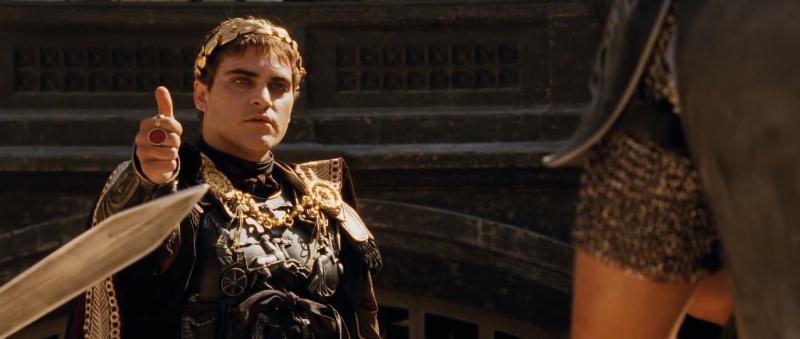This image from the movie "Gladiator" prominently features the emperor giving a thumbs-up gesture. His head is adorned with a gold laurel leaf crown, and he has short brown hair. He is dressed in black armor coupled with an opulent gold-detailed cape that drapes around him. Notably, he wears two rings on his right hand: one is a plain gold ring on his pointer finger, and the other, on his middle finger, has a gold border with a striking red circular center. At the forefront of the image, the tip of a sword emerges from the bottom right corner. On the right side of the frame, there is part of an unknown figure wearing metal armor and a green cloth, possibly a shoulder guard. The background showcases a black wall with square indentations at the top and an arched doorway with a gate. The image is wide but not very tall, providing a detailed and cinematic look into the scene's setting and characters.